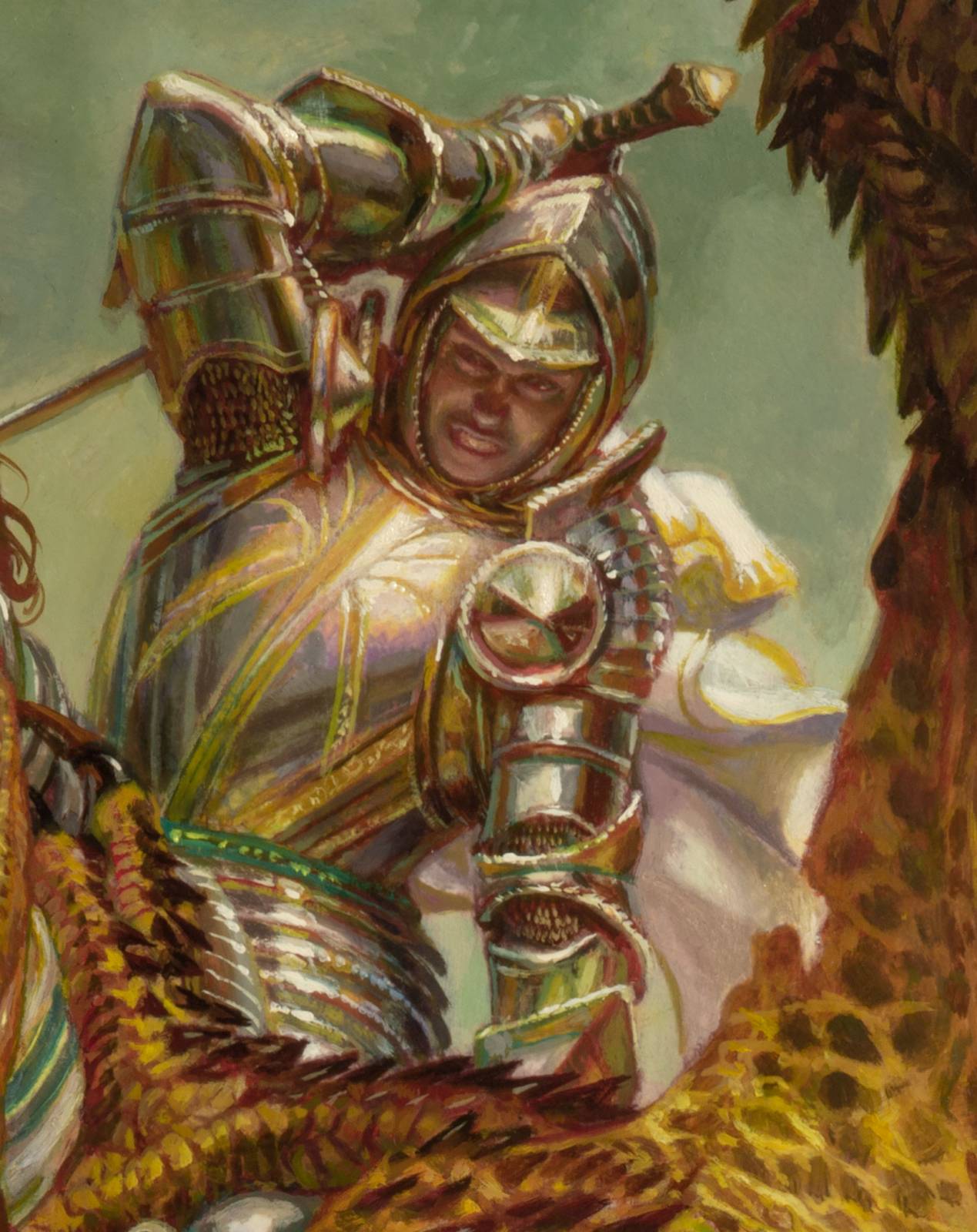This detailed digital painting illustrates a knight or paladin clad in glimmering, ornate golden armor. With his faceplate lifted, his expression shows a determined grin as he raises a large sword high above his head with his right arm, poised to strike. The knight's armor showcases a dazzling chest plate adorned with a golden, firework-like design that explodes with shimmering details. Behind him, a white cloak with gold trim flutters dramatically in the wind. In front of the knight, partially visible, is the leg of a colossal dragon, its scales a mix of brown, yellow, and black spines, hinting at an epic battle. The greenish hue of the background adds an ethereal atmosphere to the scene, contrasting with the vivid colors of the knight and the dragon. No other figures or writings are present in the illustration.